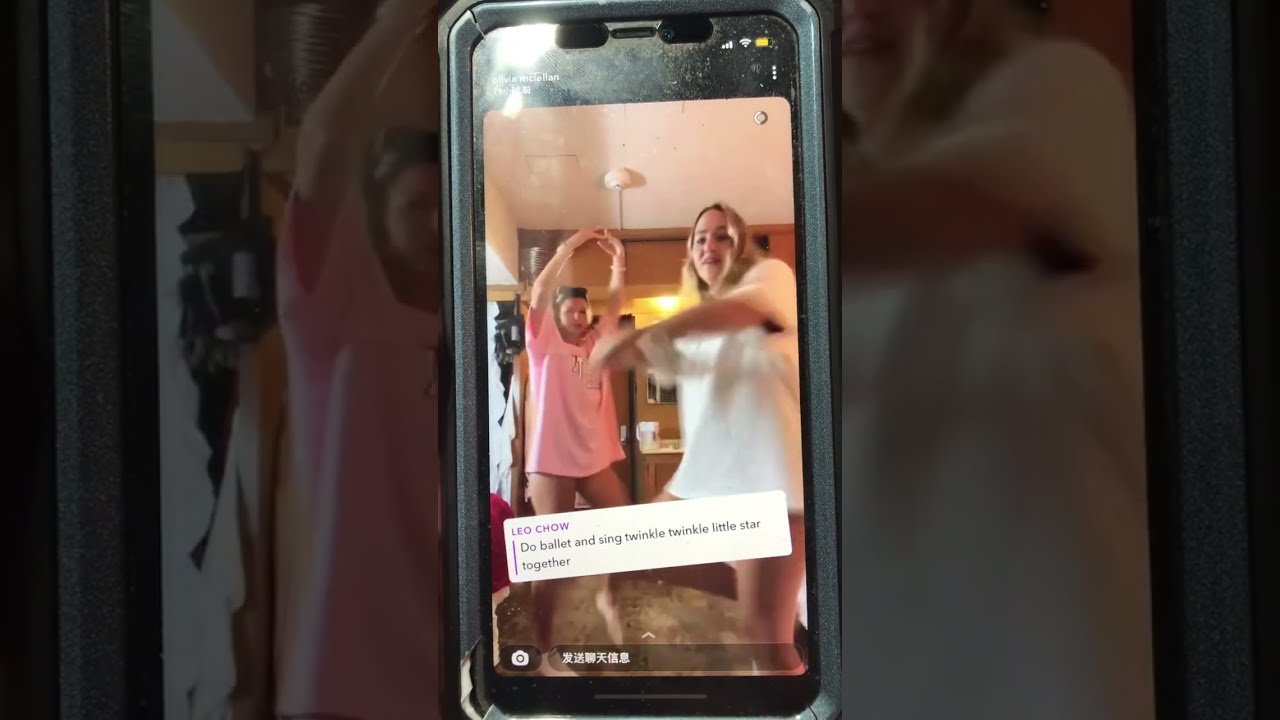This is a color photograph featuring a cell phone displaying an image of two women dancing. The cell phone has a large, thick, black case, possibly resembling an OtterBox, with two speakers visible at the top. The women in the image both have blonde hair. The woman on the right is wearing a long, white short-sleeved shirt that covers her legs, while the woman on the left is dressed in a pink short-sleeved shirt. Both women appear to be engaged in a ballet pose; the woman on the right has her arms out in a circular motion, while the woman on the left has her arms arched above her head and one foot lifted off the ground. The background of the image within the phone features a brown wall and a white wall above it, set against a brown floor. Below the dancers, there is a white banner with purple text that reads "Leo Chao" and black text below it that states, "Do Ballet and Sing Twinkle, Twinkle Little Star Together." The foreground image is also repeated in an enlarged and darkened fashion on either side of the phone, showing the detailed images of both women. A small camera icon and a clear box with text in Asian characters are also visible on the screen.